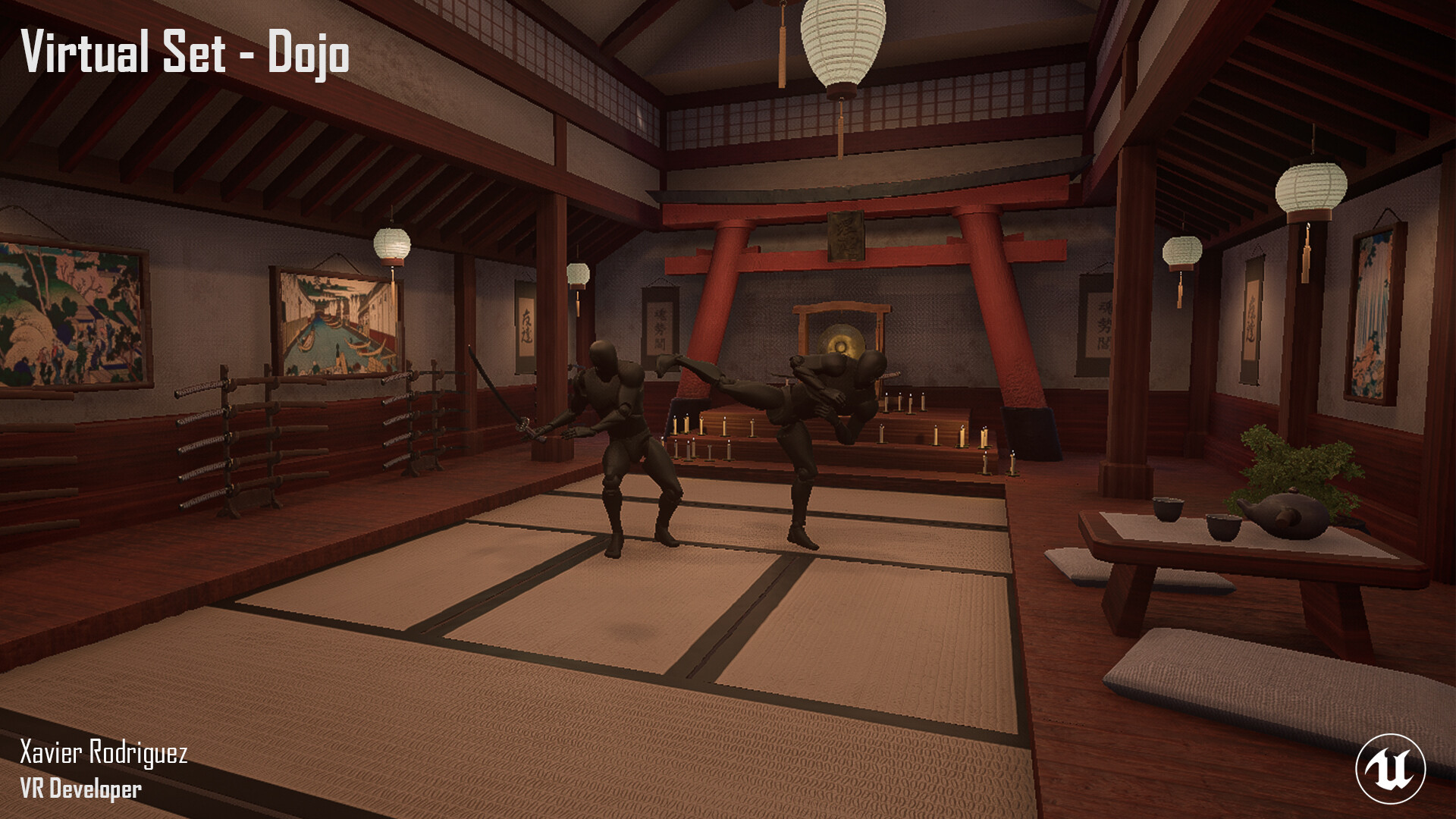The image is an in-game screenshot from a VR game titled "Virtual Set Dash Dojo," as indicated by the white text watermark at the top left. Another watermark at the bottom left credits "Xavier Rodriguez," with the designation "VR Developer" in bold white text. A transparent white circle with the Unreal Engine logo, resembling a U with the left line formed like a scythe, is positioned at the bottom right.

At the center of the image, two animated figures, depicted as wooden robots, are engaged in combat on a tatami mat. The left figure wields a wooden katana, prepared to strike, while the right figure, barehanded and barefoot, extends his right leg in a missed kick. Both figures wear tight, body-sculpted dark gray or black outfits, resembling ninjas or swordsmen.

The scene is set in a room with an oriental feel, featuring tan-colored flooring with brown lines and a background wall adorned with red support structures resembling a goal post with two crossbars. The upper walls extend outwards, displaying various Asian-inspired decorations, swords, and other art. Additionally, a table with two cups and a planter is visible on the right, alongside some oval-shaped hanging lights. Overall, the room's color palette includes brown, tan, red, yellow, and white tones.